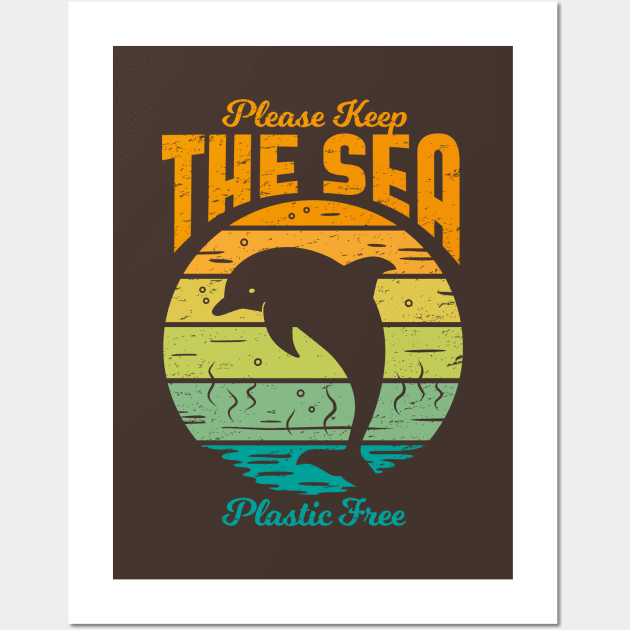The image depicts a digitally rendered poster designed for educational or social awareness purposes, situated against a light grey background with a white border. The center of the poster showcases a dark brown backdrop with a captivating composition: a black dolphin is portrayed in mid-flight, leaping out of the water. Surrounding the dolphin are stylized, multicolored wooden planks in hues of yellow, green, and blue, giving a sense of motion and depth.

At the top of the image, in a gradient font transitioning from red to blue, the message "Please Keep The Sea" is prominently displayed, arching around the circle. Below the vivid scene, at the bottom of the poster, the words "Plastic-Free" are elegantly scripted in blue cursive, emphasizing the theme of the poster. The harmonious blend of colors and detailed elements visually reinforce the call to action for maintaining a plastic-free ocean.